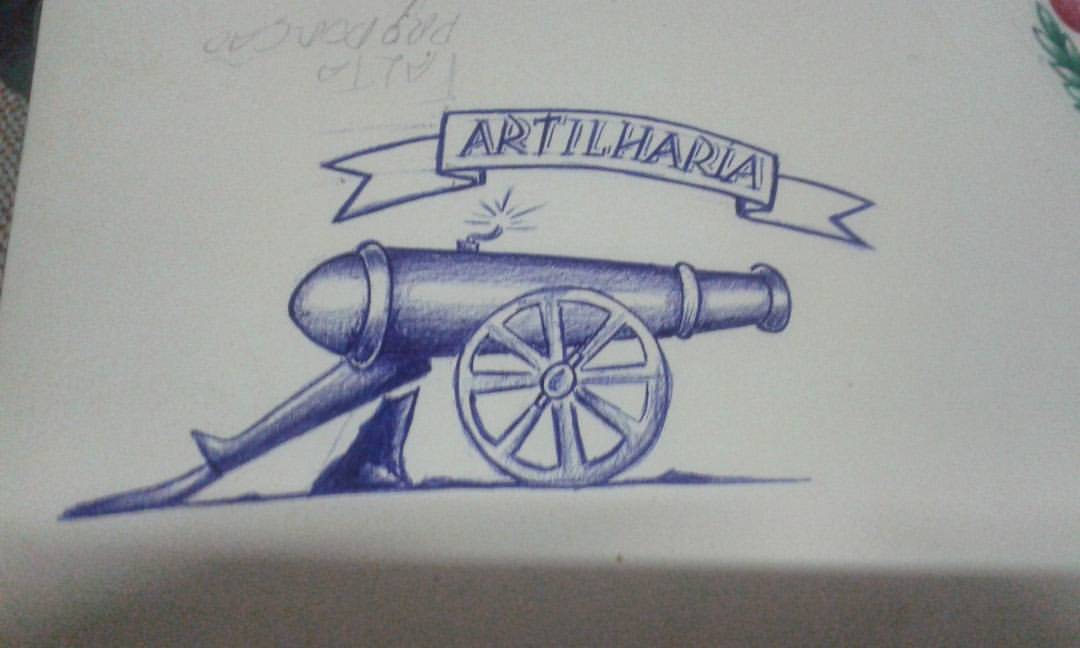This detailed drawing captures a cannon titled slightly to its side, poised to fire, with the lit wick signifying imminent discharge. The word "Artillaria" or "Artilleria" is prominently inscribed, further emphasizing the theme. The artist showcases exceptional skill and mastery over the medium, employing intricate pen shading to create depth and realism. The meticulous attention to detail highlights the cannon's texture and form, making it a striking and evocative representation of artillery.